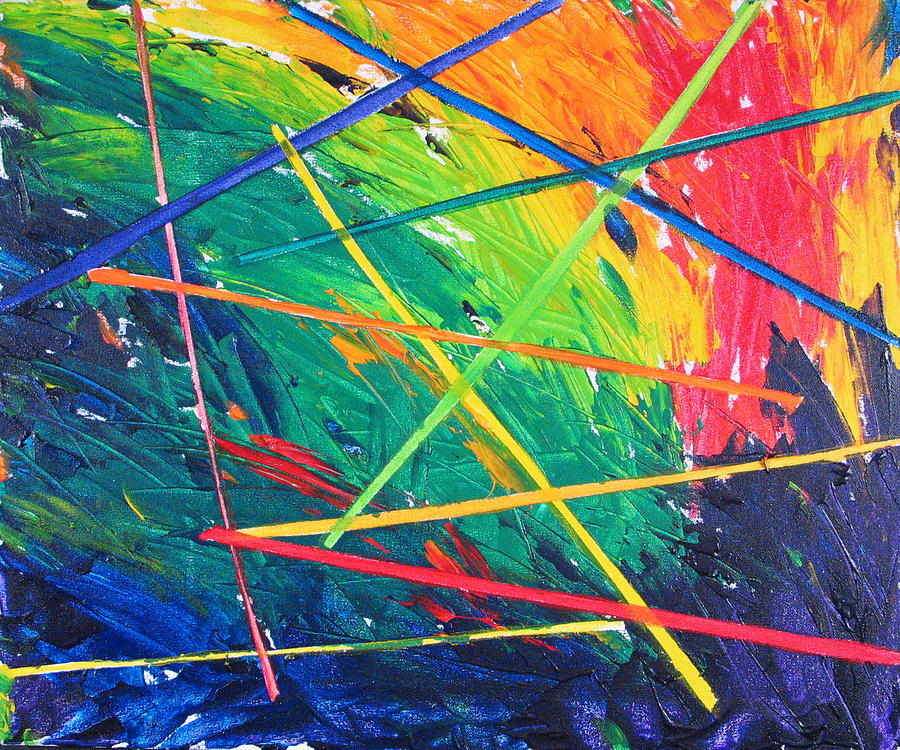This abstract painting features vibrant, rough brush strokes that overlap each other to create a dynamic and textured canvas. Starting from the bottom, a deep, dark blue extends across with smudges reminiscent of fingerprints. In the bottom left corner, hints of green and purple blend together, while the right-hand corner houses a rich, dark purple. Moving upward, a dark green emerges, transitioning into an aqua blue and a lighter shade of green above it. A stripe of light green separates these hues from an array of colors above, starting with yellow, transitioning into orange, pink, and more orange in the upper right corner. Overlaying these variegated background colors are numerous intersecting lines. Near the bottom left, a yellow line runs close to parallel, followed by a red line, an orange line, a brighter orange line, and two blue lines above them. These lines intersect with another set: blue intersecting with blue, then a yellow line crossing with a red line. The lines, varying in color from blue, yellow, red, green, and orange, crisscross in different directions—diagonal, horizontal, and vertical—adding layers of complexity to the artwork.